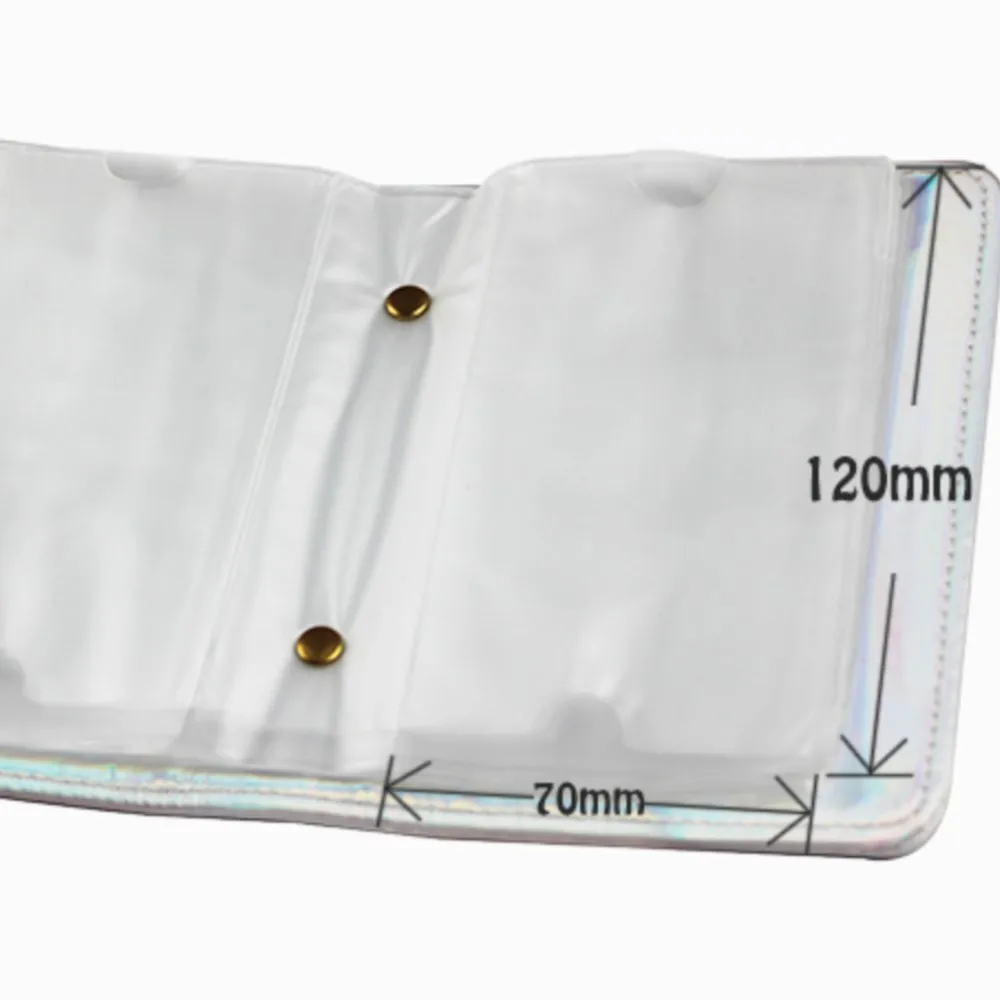The image shows a zoomed-in perspective of a white rectangular object, possibly made of fabric or plastic, set against a solid white background that makes its edges indistinct. On the right edge of the object, a vertical black arrow points both up and down, labeled "120 mm." Positioned horizontally on the object is another black arrow, marked "70 mm," extending from the right edge to about halfway across. This suggests the object might fold or be used in sections. In the center, just left of the 70 mm mark, are two shiny brass buttons or gold metal dots. These are possibly securing a flap or seam that runs across the object. The object also appears to have slight humps or elevations on both the left and right sections. Threads can be seen along the seams, indicating stitching.